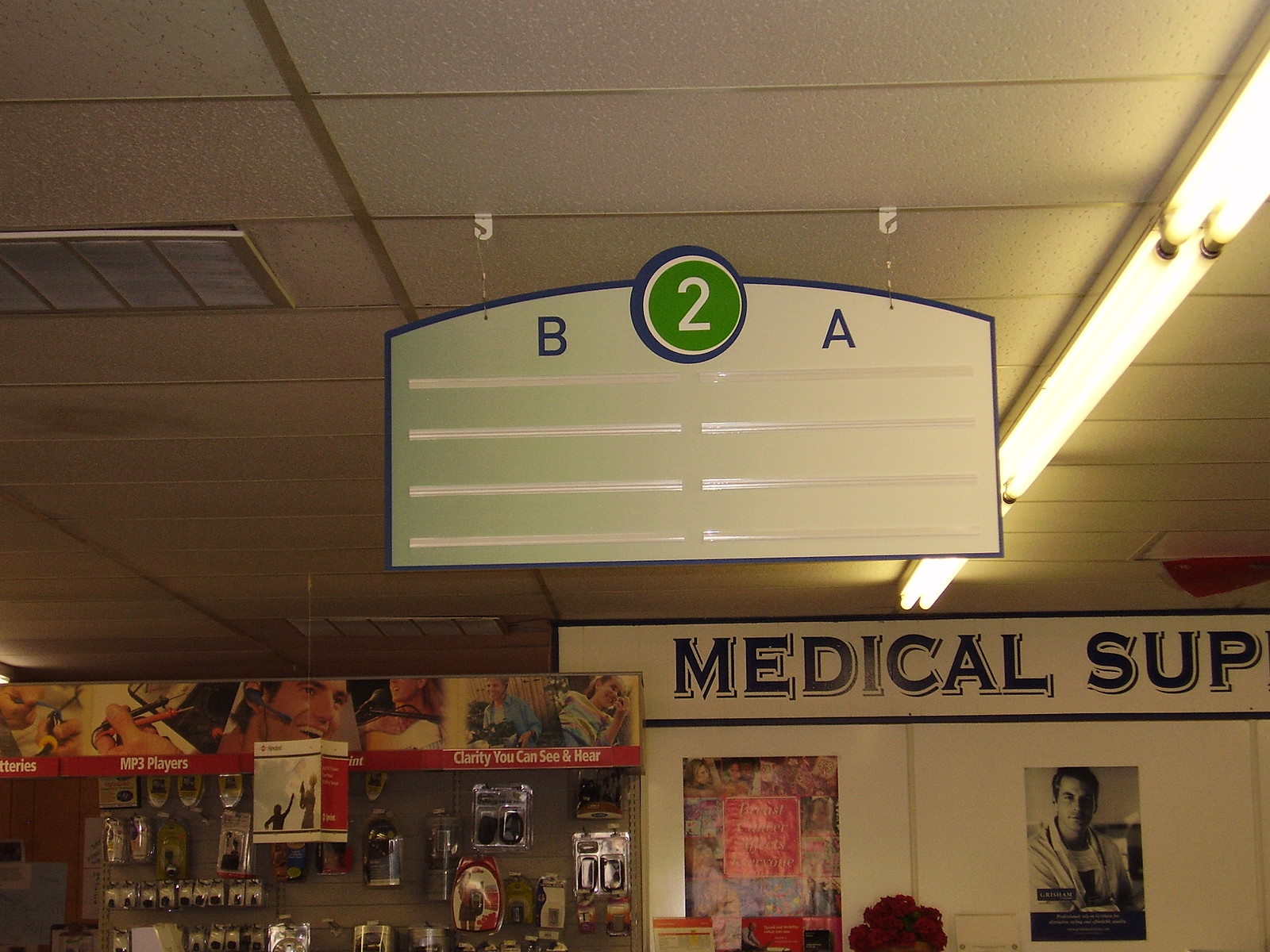This image shows the dimly lit interior of a possibly outdated general store with ceiling tiles and fluorescent lighting. A prominent white sign with a blue outline hangs from the ceiling, displaying the letters B and A on either side of a green circle containing the number 2. On the left side of the store, a section bannered with "MP3 Players" showcases various electronic accessories including MP3 players, headphones, batteries, and computer mice. These items are encased in plastic and neatly hung from the display. On the right side, a partially visible sign that reads "Medical SUP" suggests medical supplies, accompanied by an image of a doctor. Additionally, there are red flowers and what seems to be a poster with a collage of magazine cutouts. The overall ambiance and product selection hint that the photo likely dates back to the early 2000s.